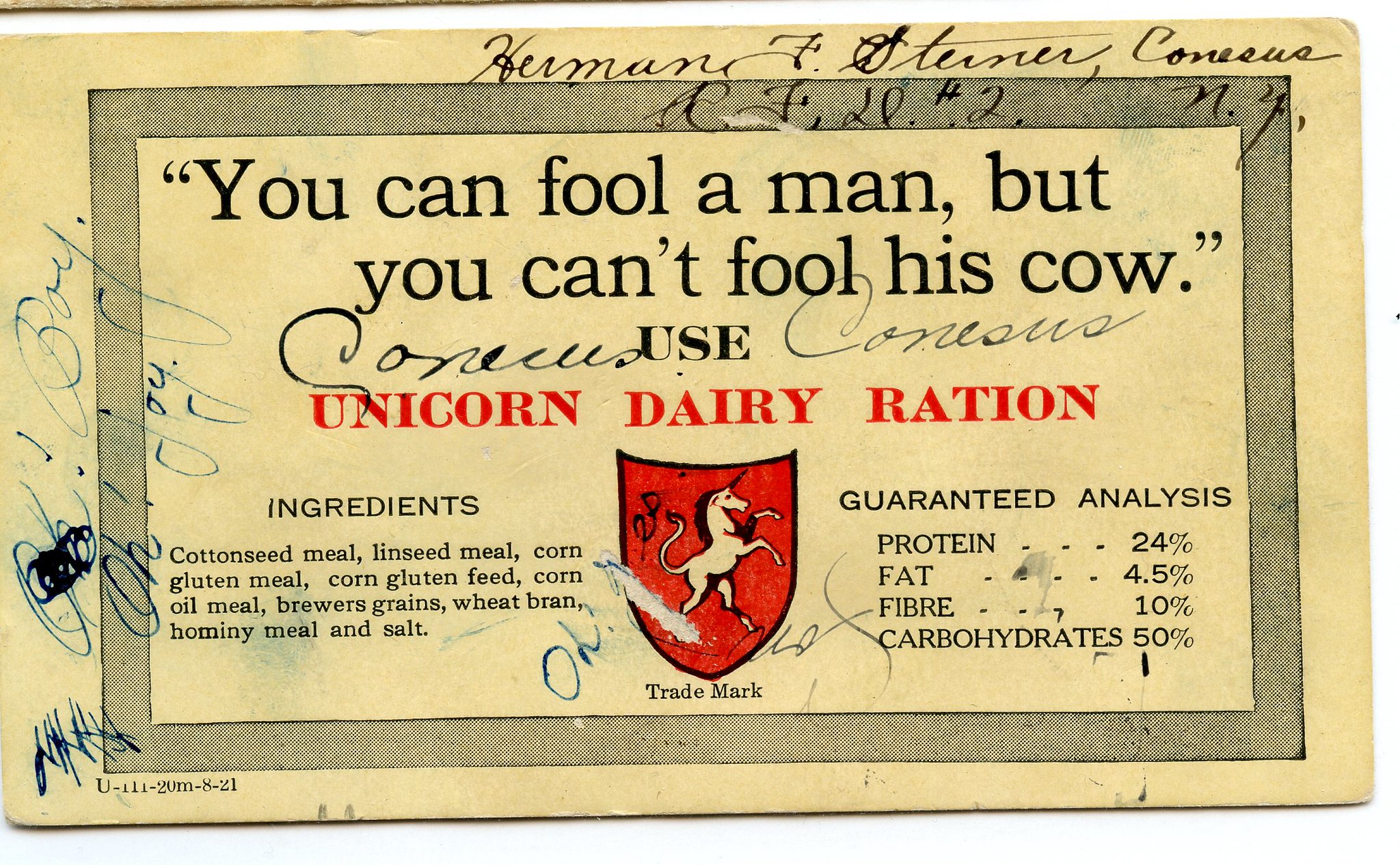This image depicts an old, tattered rectangular advertisement or note card with a beige to white background, featuring a prominent slogan in black ink: "You can fool a man, but you can't fool his cow. Use Unicorn Dairy Ration." The slogan is accompanied by a shield-shaped logo with a red background and a white unicorn. Below the logo, it states "trademark." 

To the left, the card details the ingredients: cottonseed meal, linseed meal, corn gluten meal, corn gluten feed, corn oil meal, brewers grains, wheat bran, hominy meal, and salt. On the right, it lists the guaranteed analysis: protein 24%, fat 4.5%, fiber 10%, and carbohydrates 50%. 

Both sections are surrounded by various scribbling in black and blue ink, with repeated phrases such as "oh boy" and "oh joy," making the text somewhat difficult to read. The card appears worn with obvious rips and tears, suggesting it has been handled frequently over time. Overall, the intricate details and memorable slogan create a vivid image of a vintage dairy product advertisement.